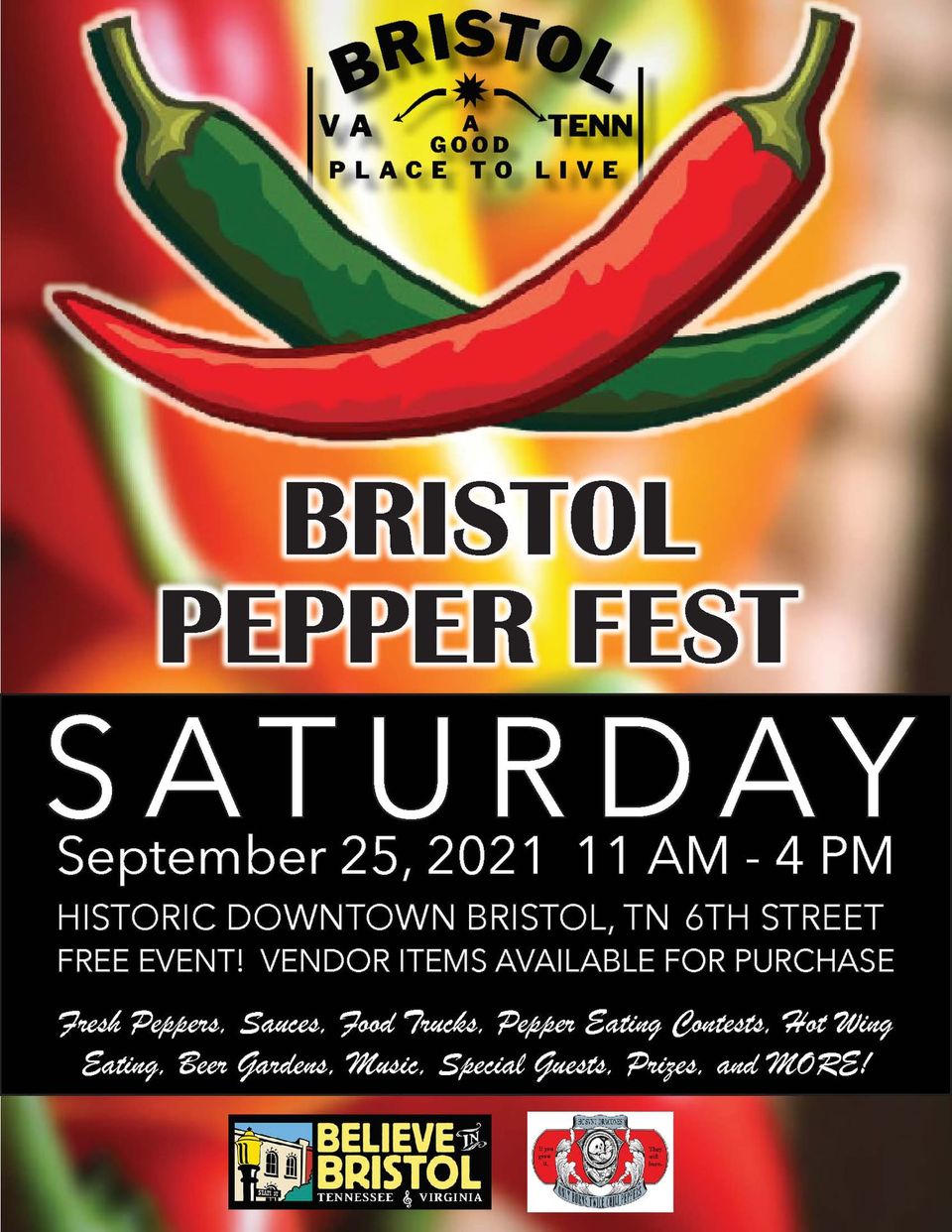The image is a detailed poster advertising the Bristol Pepper Fest. At the top, in black writing, it reads "Bristol, VA-TENN, a good place to live." Below this, two chili peppers—one red and one green—are crossed over each other. The main title "Bristol Pepper Fest" follows. Beneath this, a black banner with white font provides event details: "Saturday, September 25th, 2021, 11 a.m. to 4 p.m. Historic Downtown Bristol, Tennessee, 6th Street. Free event. Vendor items available for purchase." Further down, the poster lists event attractions, including "fresh peppers, sauces, food trucks, pepper eating contests, hot wing eating, beer gardens, music, special guests, prizes, and more." At the very bottom, it says "Believe in Bristol, Tennessee and Virginia," accompanied by some designs and two indistinct logos. The background features a blurred, colorful image of red, green, and possibly orange peppers, contributing to the vibrant chili-themed design.